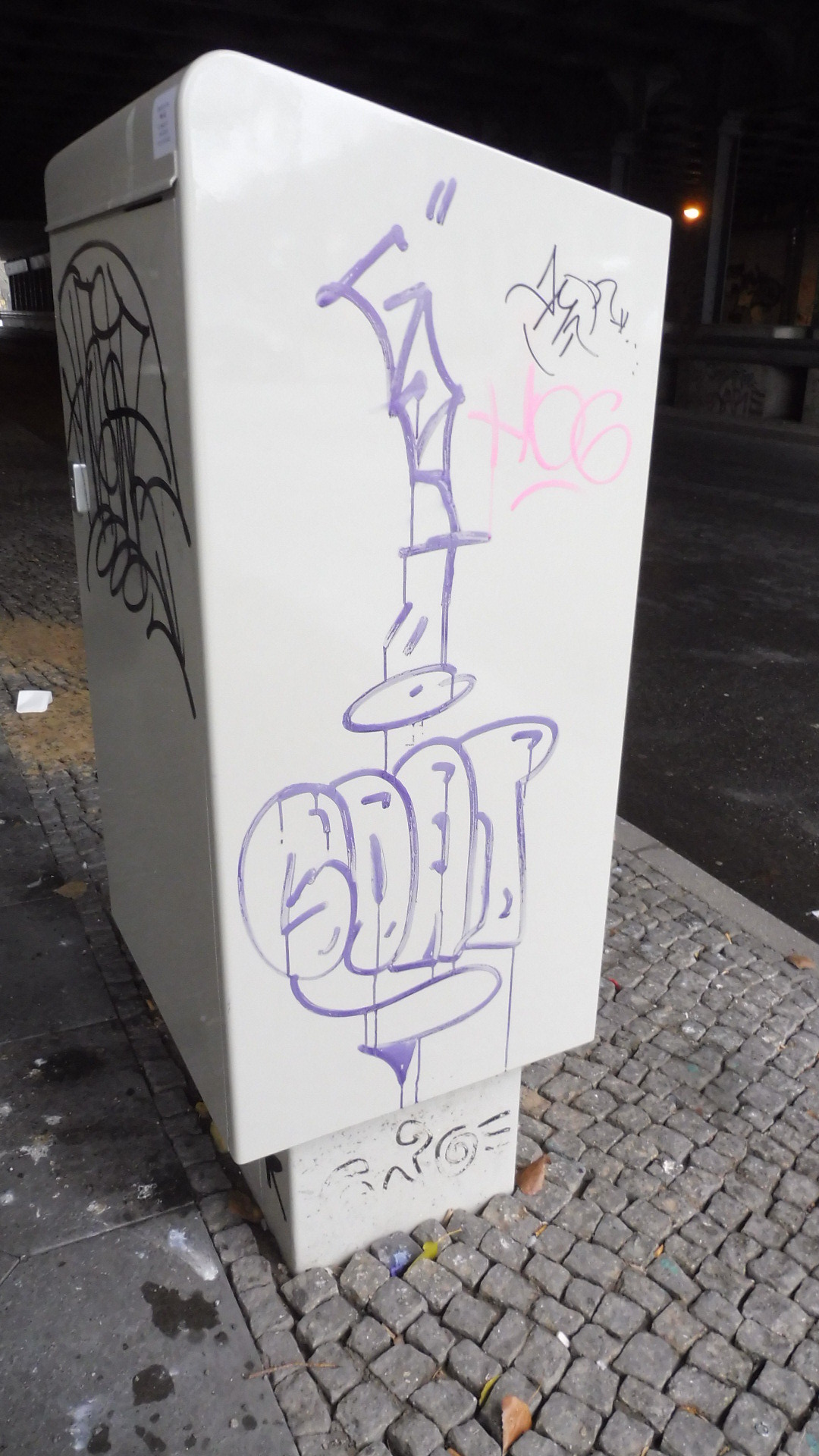The photograph captures a white, rectangular metal box, possibly an electrical or postal box, situated on a city sidewalk with cobblestone paving. Taken at night, the image reveals the contrasting darkness of the background. The box, positioned slightly to the left, is heavily adorned with graffiti, including "GOAT" in bold, bubble letters towards the bottom, and additional random lines and scribbles in black, purple, and pink hues. On the front, near the handle of the door, more graffiti in black marker is visible. Scattered trash around the base of the box further highlights the area’s neglected state.